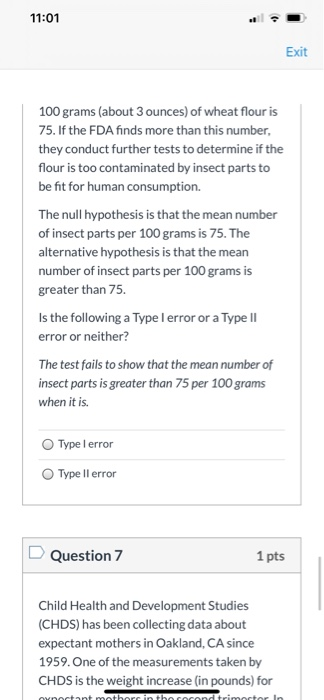A detailed image caption:

The image is a screenshot taken from a mobile device, displaying the time as 11:01 and a battery level of approximately 85% at the top of the screen. The top of the image features a blue "EXIT" button. The main content describes a statistical problem related to wheat flour contamination by insect parts as per FDA guidelines. The text explains that 100 grams (about 3 ounces) of wheat flour should contain no more than 75 insect parts, and if this threshold is exceeded, further testing is required to determine its suitability for human consumption. The null hypothesis states that the mean number of insect parts per 100 grams is 75, while the alternative hypothesis proposes that it is greater than 75. The question posed is whether a test that fails to show the mean number of insect parts exceeds 75 per 100 grams, when it actually does, constitutes a Type 1 or Type 2 error, or neither. At the bottom, there are options to select Type 1 error or Type 2 error, and the question is labeled as "Question 7."